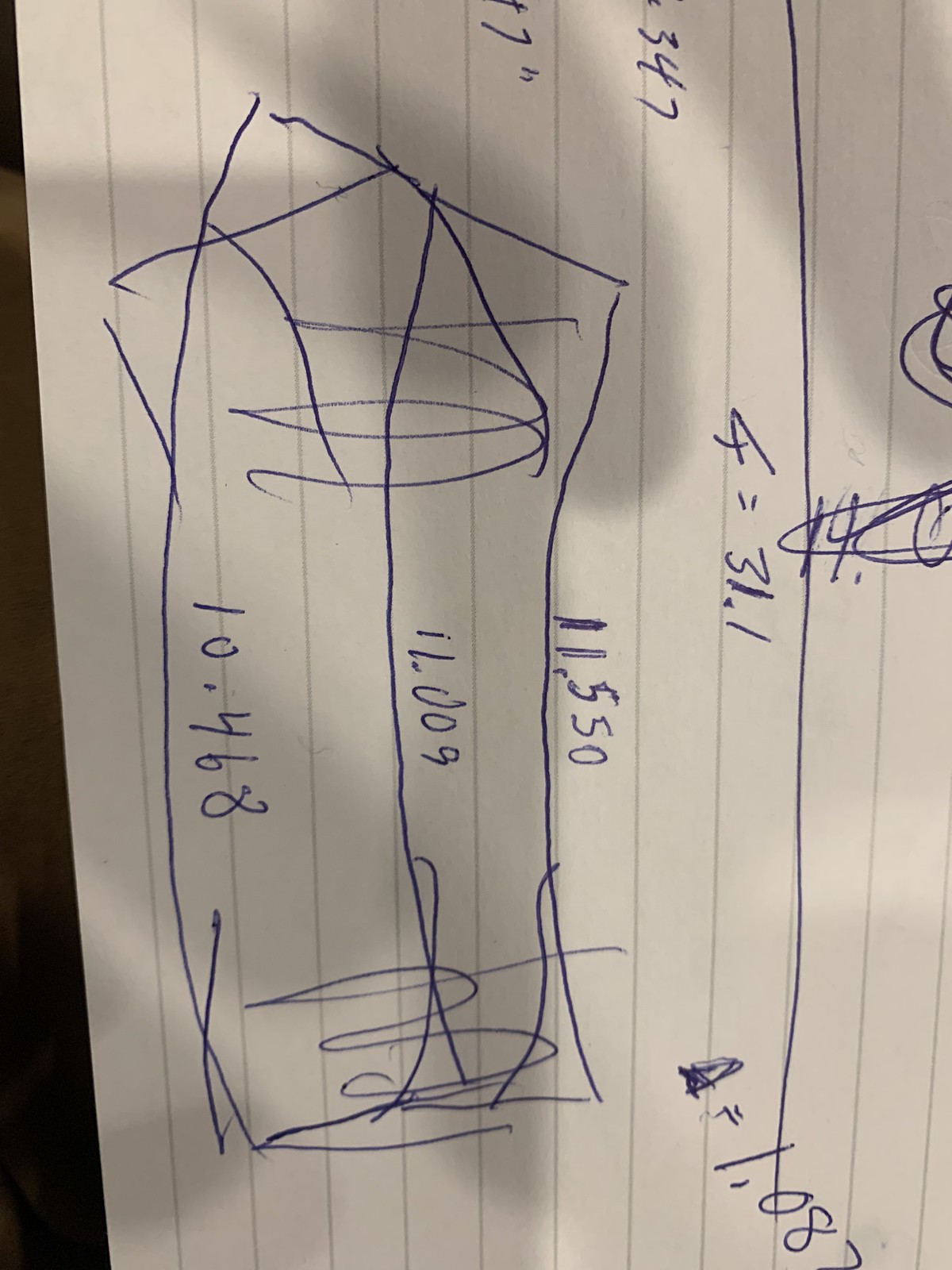The image displays a piece of notebook paper oriented sideways, causing the lines to run vertically instead of horizontally. The left edge of the image reveals a narrow strip of an indistinct brownish background. The paper itself is marked up with various blue pen markings. In the bottom right corner, there's a notation "A = 1.087." Adjacent to it, there's a less-than symbol crossed by a slash, followed by "= 31.1." Near this, a number "14" is scribbled through. 

A straight blue vertical line intersects these annotations. Further marking the paper are three vertical, slightly curved lines that form a rectangular shape, containing squiggly circles at their top and bottom intersections. The lines bear numeric values on the right-most line: "11.550," followed by "11.009" on the next inward line, and "10.468" on the innermost line.